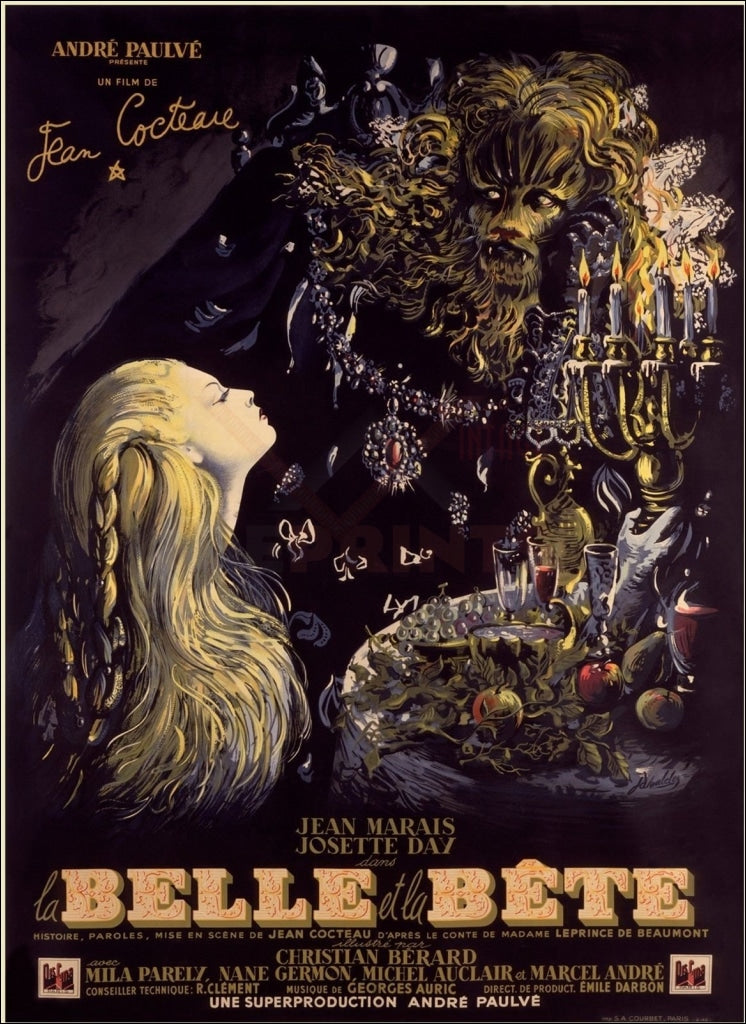This is an illustrated, old-fashioned movie poster for a French production of "Beauty and the Beast," presented by André Pavé and directed by Jean Cocteau. In the top left corner, gold text reads, "André Pavé presents un film de Jean Cocteau." The poster features two main characters: in the top right, a regal figure with a cat-like face, a flowing gold mane, and an ornate silvery chain adorned with a red gem, indicative of the Beast; and in the bottom left, a beautiful young woman with long, flowing blonde hair, partially braided and pulled back, representing Beauty. The bottom right of the poster showcases a lavishly set table with various gold and silver glasses, containers, and a large gold candelabra with five lit candles. At the bottom, additional gold text lists names associated with the production: Christian Bérard, Mila Parély, Jean Marais, Michel Auclair, and Marcel André. The entire design exudes an air of vintage elegance and fantasy.